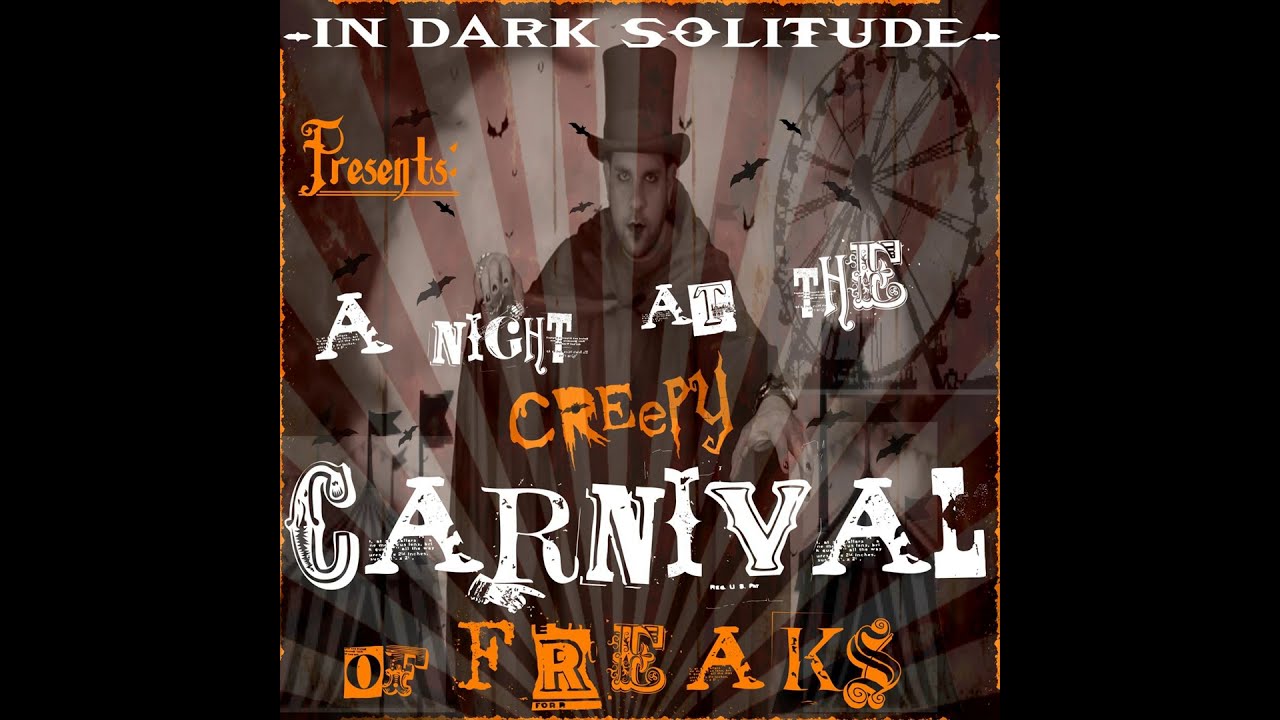The image is a rectangular, color photograph, reminiscent of an advertisement or a poster, with black sidebars approximately an inch and a half thick on each side, framing the content. Centered within these borders, the image measures roughly four inches by four inches. The topmost part features the text in white and orange typography. Starting with "In Dark Solitude" in white, it transitions to orange for "presents," back to white for "a night at the," then orange for "creepy," white for "carnival," and concluding with orange for "of freaks." This sequence reads as: "In Dark Solitude presents a night at the creepy carnival of freaks."

Central to the image is a sinister magician, adorned in a black robe and a top hat, with dark fingernails, a five o'clock shadow, and theatrical makeup, giving him an ominous appearance. Surrounding him are various eerie elements: several bats flit around him, while the backdrop features red and white stripes suggesting a circus tent. The silhouette of a Ferris wheel is visible over his left shoulder, and circus flags are positioned to his right, adding to the carnival atmosphere.